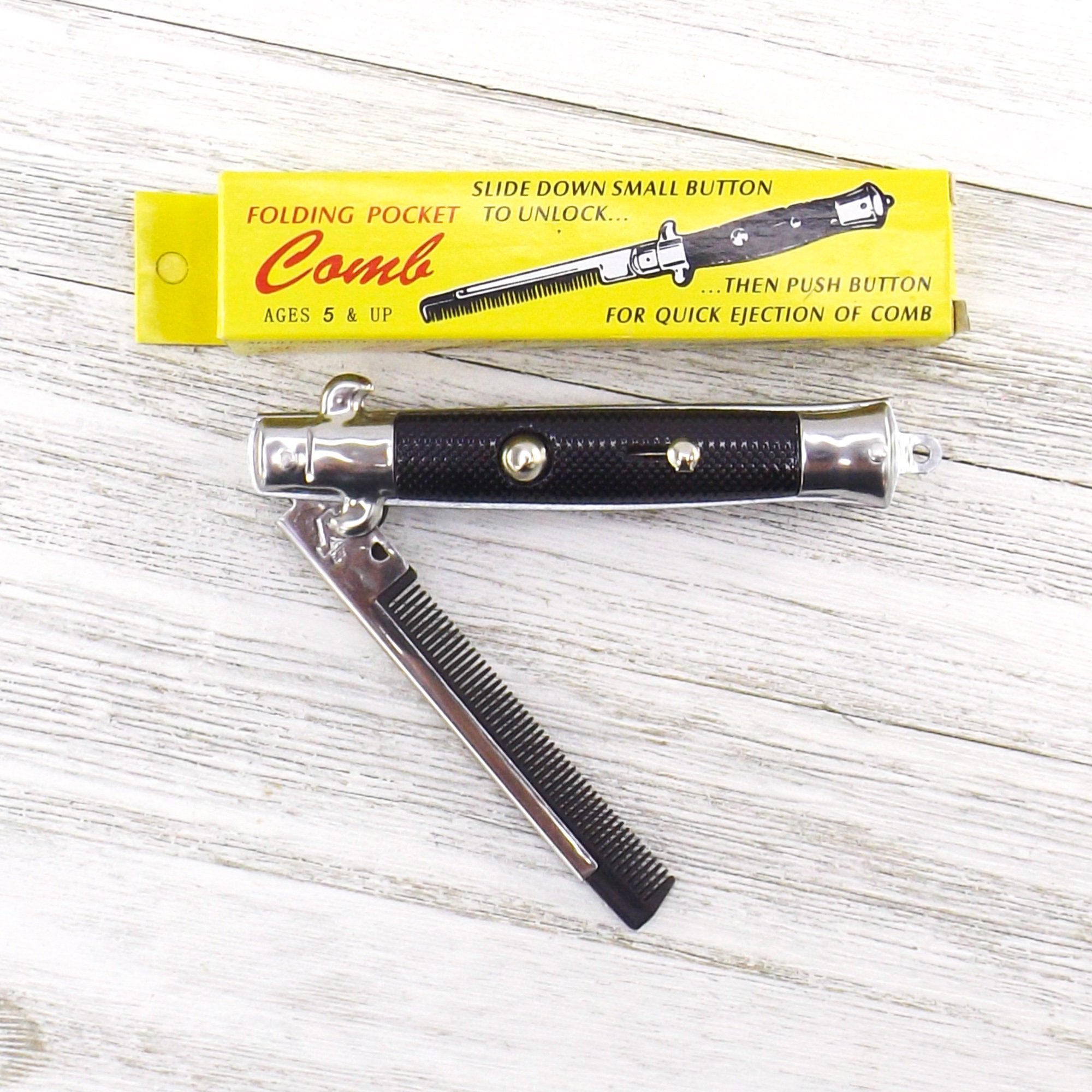This overhead photograph captures a folding pocket comb and its packaging on a white-painted wooden table with visible wood grain. The comb, designed to resemble a switchblade, features a black handle with silver tips and an extended black comb. The comb is partially opened, creating an inverted V shape with the mouth pointing toward the bottom right corner of the image. Above the comb lies its yellow box, oriented vertically, measuring approximately three to four inches in length. The packaging prominently displays "Folding Pocket Comb" in red script and below that, "ages five and up" in smaller black text. An illustration of the fully extended comb is shown on the box, with accompanying instructions: "slide down small button to unlock" above the illustration and "then push button for quick ejection of comb" below it. The box also features additional three-dot lettering in the bottom right corner.